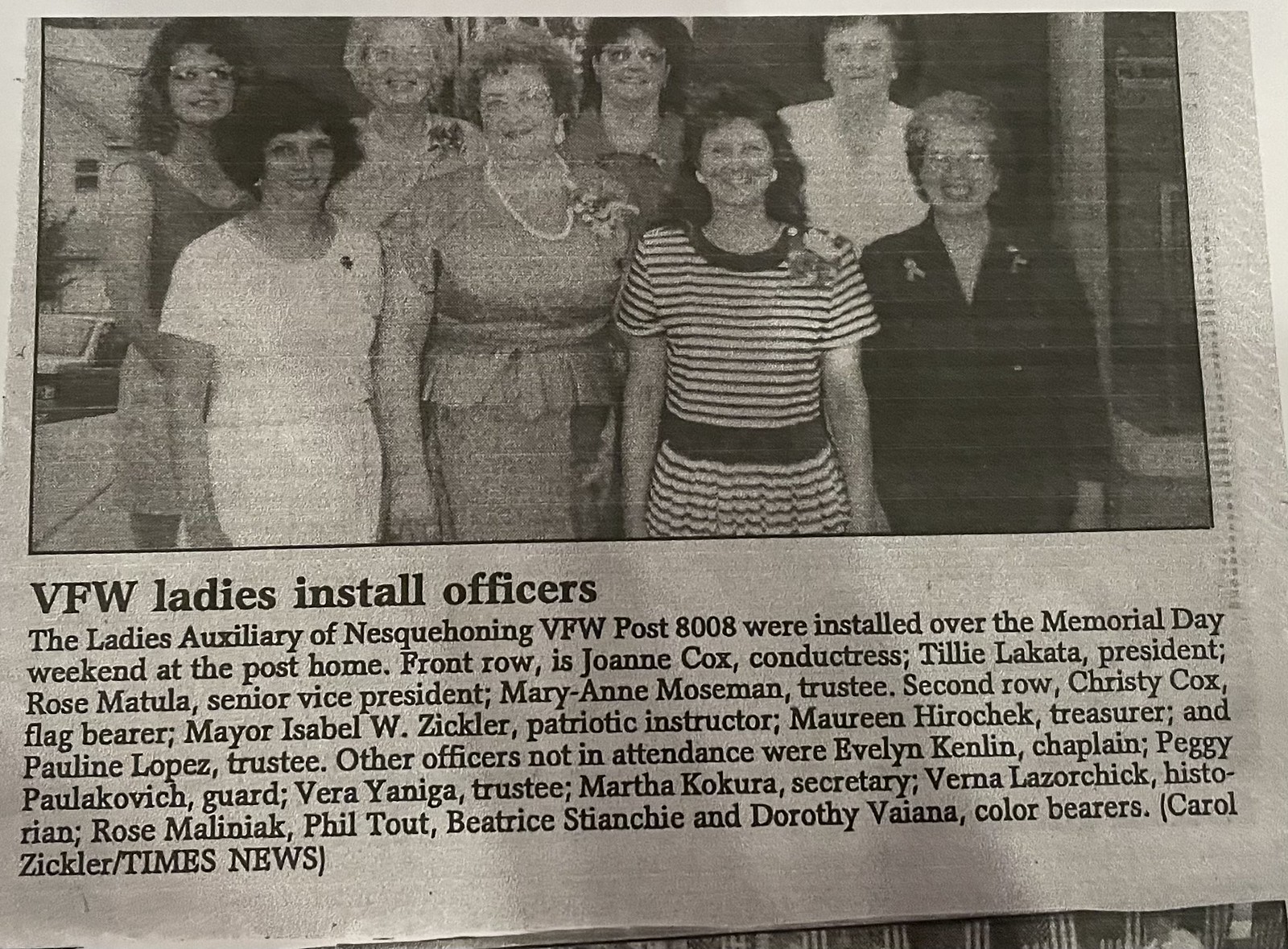The image is a photograph of an old newspaper clipping, which is rectangular and wider than it is tall. At the top, occupying about two-thirds of the clipping, is a black-and-white photograph showing eight women posing for a picture in front of a house. They are arranged in two rows, with four standing in the front and four behind them. Below the photograph, bold text reads "VFW Ladies Install Officers," and the detailed caption explains that the Ladies Auxiliary of Nesquehoning VFW Post 8008 were installed over the Memorial Day weekend at the post home.

The individuals in the front row are identified as Joanne Cox, Conductress; Tilly Licata, President; Rose Matula, Senior Vice President; and Mary Ann Moseman, Trustee. In the second row are Christy Cox, Flag Bearer; Mayor Isabel W. Zickler, Patriotic Instructor; Maureen Herochek, Treasurer; and Pauline Lopez, Trustee.

Additionally, other officers not in attendance are listed: Evelyn Kenlan, Chaplain; Peggy Polakowicz, Guard; Vera Yaniga, Trustee; Martha Kukura, Secretary; Vera Lazarczyk, Historian; Rose Melaniuk, Phil Tout; Beatrice Sianci; and Dorothy Vaina, Color Bearers. The caption concludes with "(Carol Zickler, Times News)." 

This comprehensive caption captures the essence of the photograph and the historical significance of the event it documents.